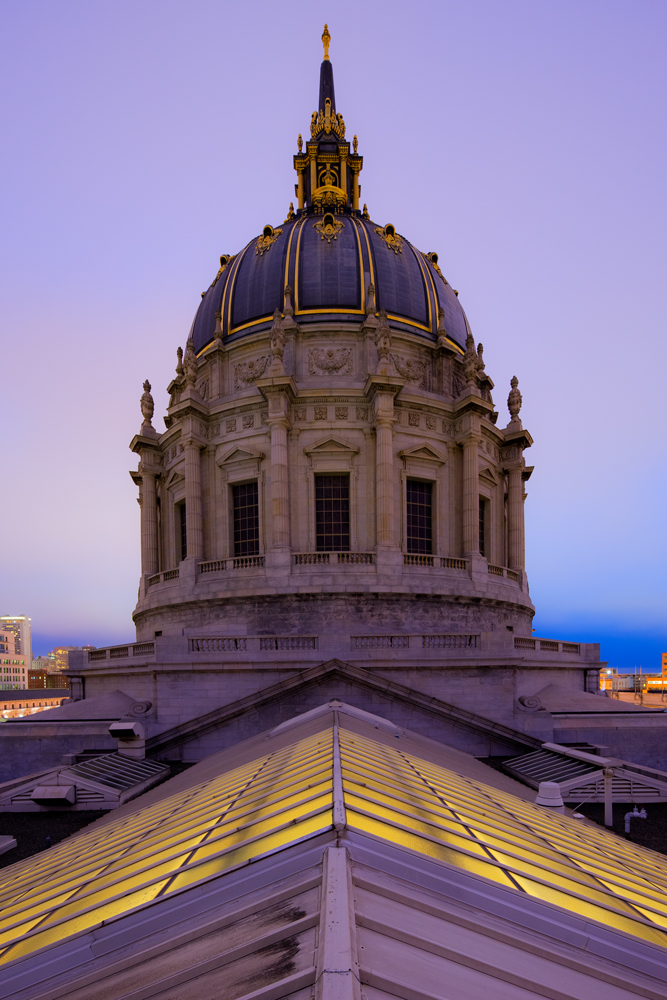In this stunning photograph, the central focus is a magnificent circular building, possibly a religious structure, distinguished by its grandiose dome. The dome is adorned with intricate gold-outlined panels and crowned with an elaborate pinnacle featuring more golden details and figurines, culminating in a blue spire topped with a golden finial. 

The image is set against a mesmerizing backdrop of a twilight sky, which transitions from a darker blue at the bottom to a vivid purple, creating an enchanting contrast. The cityscape extends into the distance, providing a sense of scale and context. 

In the foreground, there's a platform area encircling the dome, bordered by sturdy railings that hint at a walkway for visitors. Additionally, the top of an adjacent building is visible, showcasing a roof constructed from glass panels that emit a warm, inviting light from within, adding depth and intrigue to the overall scene.